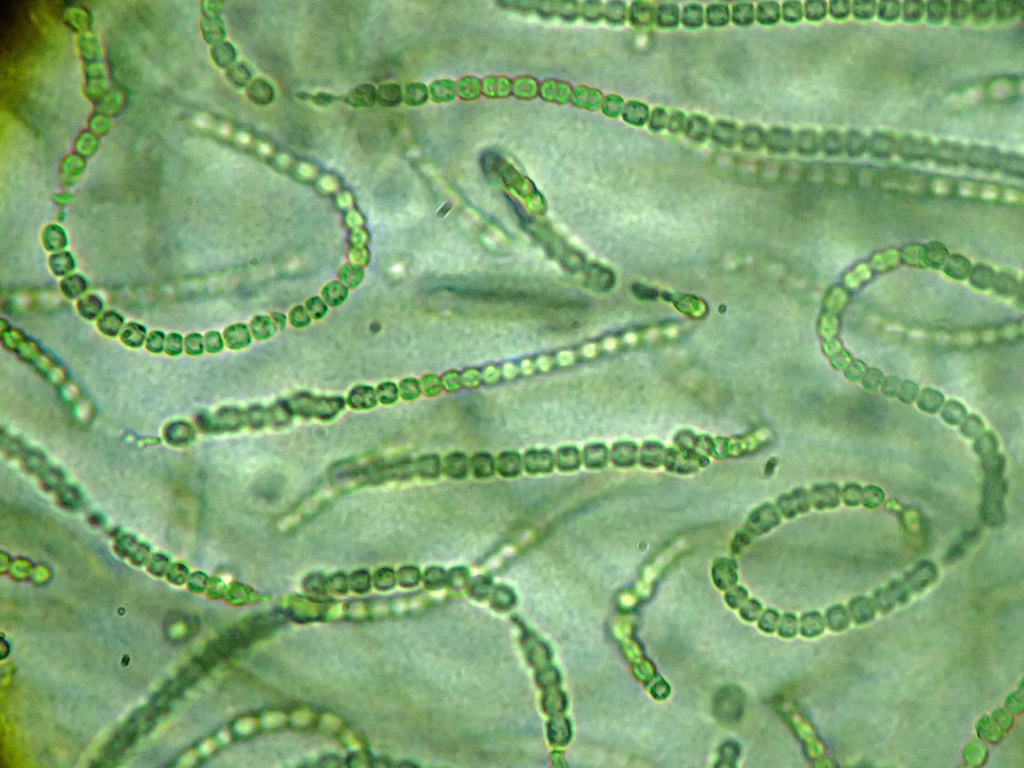This image captures a magnified view of microorganisms under a microscope, featuring a predominantly green color palette. The organisms are composed of small bead-like segments, varying in shape and arrangement. They appear as green dots or circles of different shades, close together and linked in a chain-like format. Notably, at the upper left, there is a loop-shaped chain, while an S-shaped chain is situated on the right-hand side. The top section shows a chain running horizontally from left to right, and there are areas where some chains crisscross, particularly in the bottom left. The backdrop has a slight haze, contributing to an overall older and slightly blurry aesthetic. This detailed snapshot resembles looking through a petri dish, with white areas visible where the green organisms are not present.